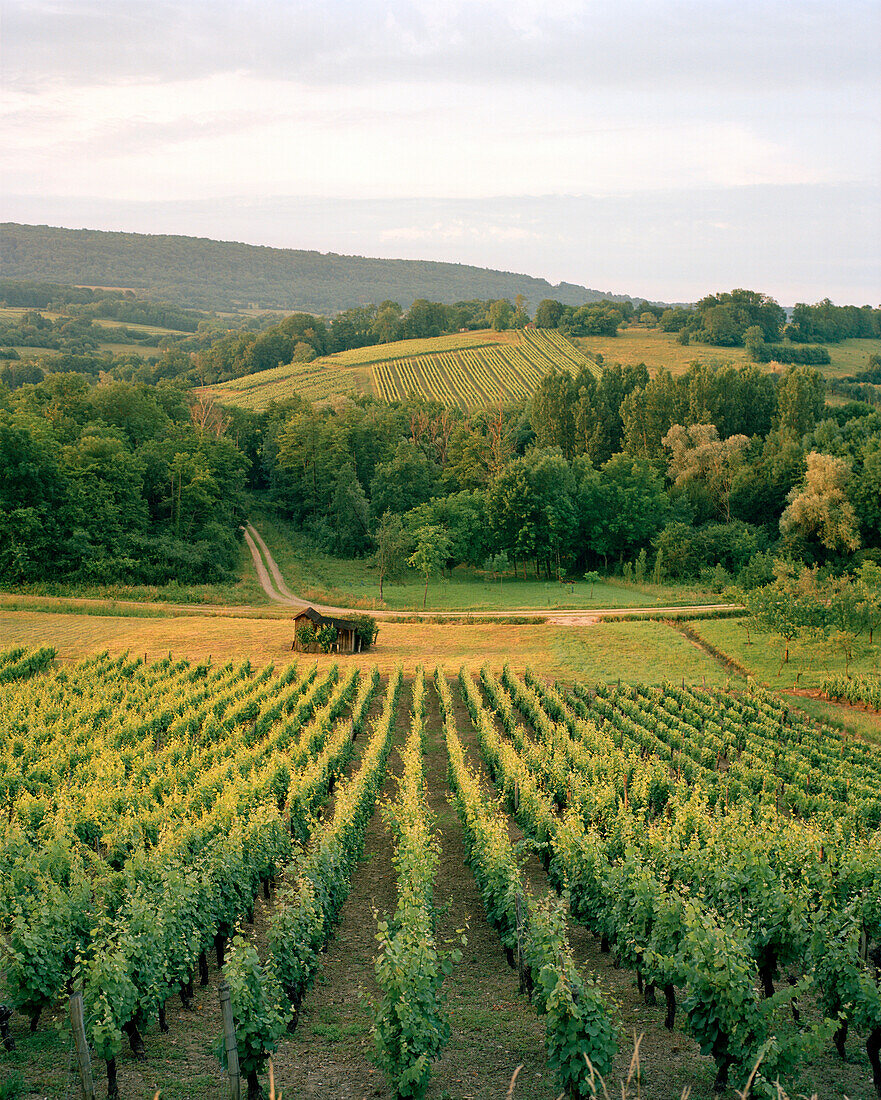This detailed image captures a sprawling farming landscape set under a mixed sky, transitioning from gray to a light blue with white, wispy clouds. Rolling hills and fields stretch across the landscape, interspersed with areas of dense trees. Most prominent are the numerous fields, some planted with green crops and others with rows of yellow-flowered plants, possibly fruit trees. In the foreground, neat rows of crops are visible, well-defined against the soil. The countryside scene is rich with textures and colors, featuring hills that recede into a distant small mountain range. 

Toward the center of the image, nestled in a small valley or depression in the landscape, lies an abandoned shed. This brown, wooden structure, with a black roof, is surrounded by a sparse cluster of three trees and sits on a patch of dry, brown grass, highlighting its abandonment. Nearby, an empty brown field gives way to other agricultural plots. A road runs horizontally across the middle of the scene, intersected by another road that vanishes into a tree line, adding depth and structure to the composition.